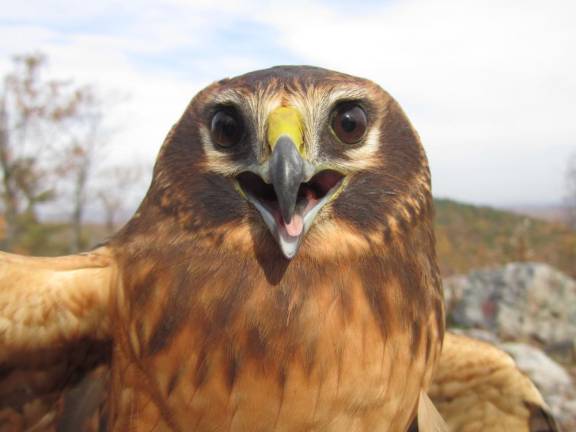This close-up, square-shaped photograph captures a detailed image of a bird of prey, likely a hawk. The bird is shown from the upper breast up to the head, positioned head-on and staring directly into the camera. Its beak is slightly open, revealing a visible tongue, and features a yellow bridge extending across it, transitioning to a gray tip. The hawk's piercing brown eyes are surrounded by lighter feathers, which contrast with the darker brown feathers on the top of its head and cheeks. Its plumage displays a striking array of tawny, orange, and beige colors, with the wings slightly spread out to the sides, connecting to the torso. In the background, some foliage, likely trees or bushes, extends from the left side of the image, with a hilly terrain featuring grasses and rocky outcroppings. The leaves on the trees indicate a season of early fall, showcasing a blend of green and reddish hues. The sky appears mostly cloudy with patches of blue, suggesting a clear yet partially cloudy day. The bird's intimidating gaze and open beak add to the intensity of this arresting daytime shot.